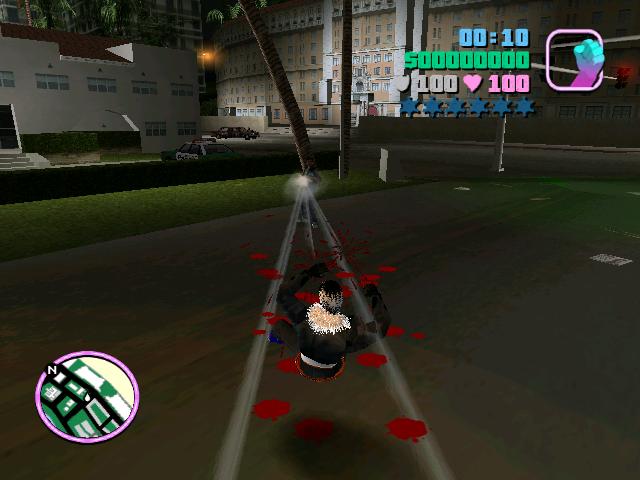A screenshot from a video game captures a character in the middle of a nighttime urban setting. The character, dressed in black with a white hood, is holding a pair of poles positioned at an angle, possibly in the process of constructing a teepee-like structure. The scene is illuminated by the surrounding buildings, and various game interface elements are visible. A timer at the top of the screen reads "00:10," which could indicate either 10 minutes or 10 seconds elapsed. The player's health is displayed as 100 hearts, suggesting they are in optimal condition. Additionally, there are star icons, whose purpose remains unclear, potentially representing achievements or collectibles. The image seems to capture a moment early in the game's progression, as indicated by the low score.